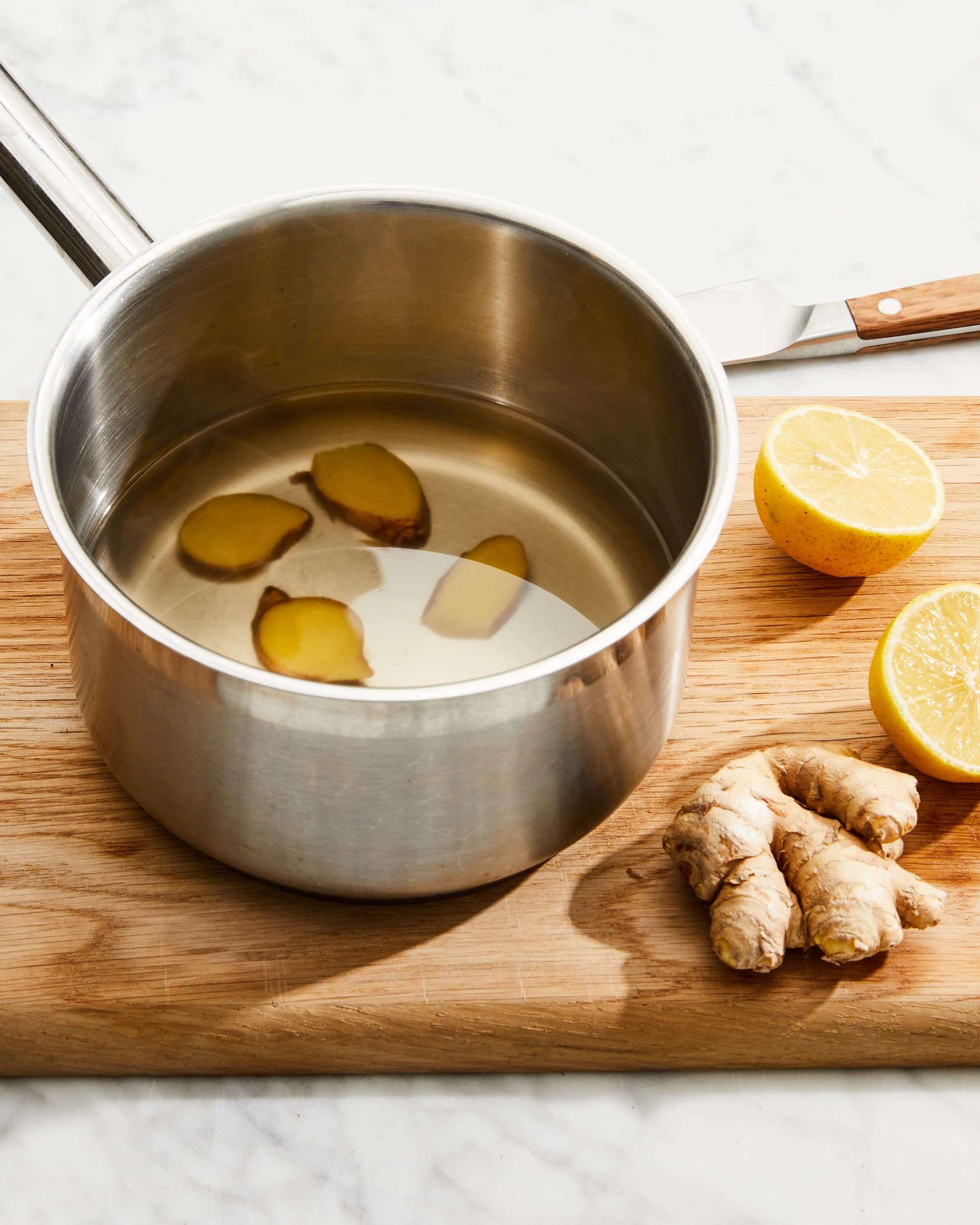On a cloudy-patterned white and gray marble countertop, a light wooden cutting board holds a small silver pot partially filled with about a quarter cup of still water. Sliced ginger pieces float in the liquid inside the pot. On the cutting board, there is also an unpeeled whole ginger root and two lemon halves lying next to the pot; one of the lemon halves has two seeds visible inside. At the back of the cutting board, a stainless steel knife with a brown wooden handle, matching the cutting board, rests partly visible. This arrangement, evocative of the beginning stages of a recipe or simmer pot preparation, showcases the neat and uncluttered look of the ingredients laid out for use.